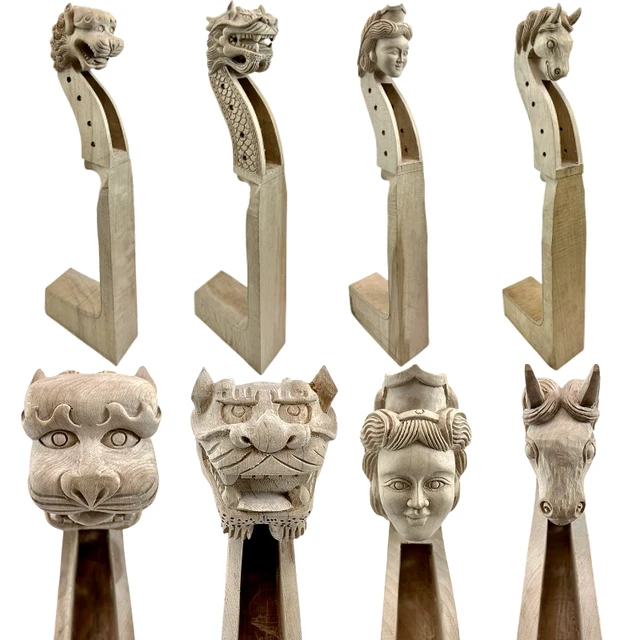In this image, we see a series of intricately carved wooden figurines set against an all-white background, creating a clean and minimalist aesthetic. The figurines, which appear to be about four in number, are arranged horizontally across the top portion of the image. Each figurine features a unique head atop an L-shaped base that resembles a checkmark, giving the objects a medieval feel. From left to right, the heads are shaped like a lion, a dragon, a woman in a crown, and a horse with two horns. The dragon's neck is adorned with textured scales, while the other figurines have smooth surfaces, each featuring four holes along their necks, possibly indicating a purpose such as threading or lacing. The figurines seem to be carved from wood, perhaps balsa wood, and the entire scene lacks any text. Dominated by neutral colors like white, tan, gray, brown, and black, the image appears as a stock photo, possibly intended for a website that sells such decorative items, which could serve as wine bottle holders or bookends. Detailed close-ups of the figurines' faces occupy the bottom section of the composition, providing a clearer view of their intricate carvings.